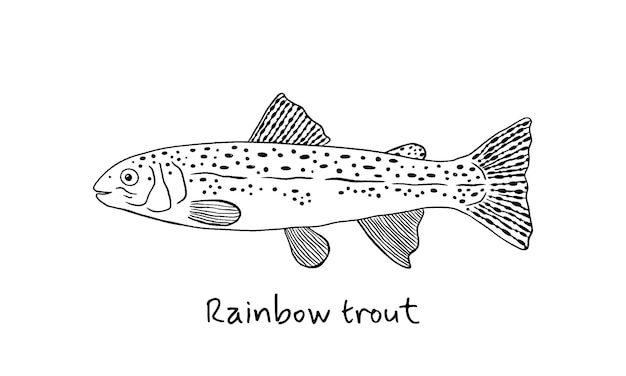This image showcases a detailed black and white drawing of a rainbow trout, set against an entirely white background. The trout is positioned facing the left, displaying a single, alert eye with a distinct white speck within its black pupil. Its mouth is open, giving the fish a lively and smiling appearance. The body of the trout is adorned with speckled black spots concentrated along the top, while the fins and tail feature prominent, elongated black lines that emphasize their shape. 

Notably, the drawing meticulously captures the trout's anatomy, illustrating the gills near the front, one side fin, two top fins, two bottom fins, and a striped tail fin. Beneath the fish, the words "Rainbow Trout" are inscribed in bold cursive writing, with the initial 'R' of "Rainbow" capitalized, and the 't' in "trout" in lowercase, adding an elegant touch to the image. This creates a cohesive, well-defined depiction of the rainbow trout, highlighting both artistic detail and biological accuracy.